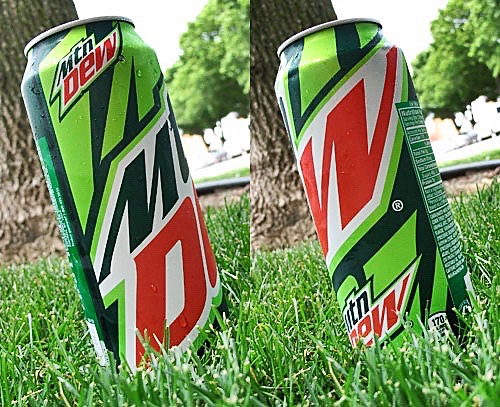A side-by-side comparison of two photographs showcases a Mountain Dew can resting on a lush, green lawn. In the left image, the can is tilted diagonally to the left, prominently displaying its iconic green, red, and white logo in a bold, eye-catching design. The background features a clear daylight sky with majestic trees and the brown bark of a tree trunk to the left, adding a natural, scenic touch to the setting.

In the right image, the can is seen from a slightly rotated angle where the nutritional information is partially visible, particularly noting "170," which likely indicates the calorie content. The detailed texture of the can's surface is highlighted, and you can also observe a portion of the label on the back. The subtle hint of morning dew on the grass adds a fresh, invigorating feel to the scene, emphasizing the refreshing nature of the beverage. Together, these photos provide a dynamic and detailed view of the Mountain Dew can in a picturesque outdoor setting.